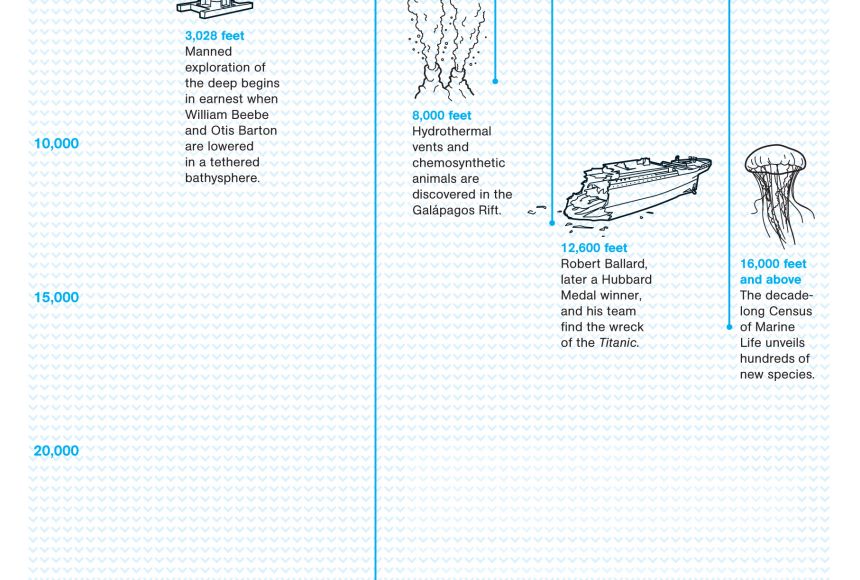This infographic, presented on a solid white background with blue patterns, illustrates various significant events and discoveries in ocean exploration, labeled with both text and icons. The left side features depth markers at 10,000, 15,000, and 20,000 feet. Despite the image being slightly cropped, key events are noted: at 3,028 feet, human deep-sea exploration began when William Beebe and Otis Barton were lowered in a tethered bathysphere; at 8,000 feet, the discovery of hydrothermal vents and chemosynthetic animals in the Galapagos Rift is highlighted; at 12,600 feet, Robert Ballard and his team's discovery of the Titanic wreck is marked with an illustration of the ship; and at 16,000 feet and above, the decade-long census of marine life that unveiled hundreds of new species is noted with an icon of a jellyfish. Arrowed lines with blue dots guide viewers through the graphic, enhancing the clarity of this detailed chart.